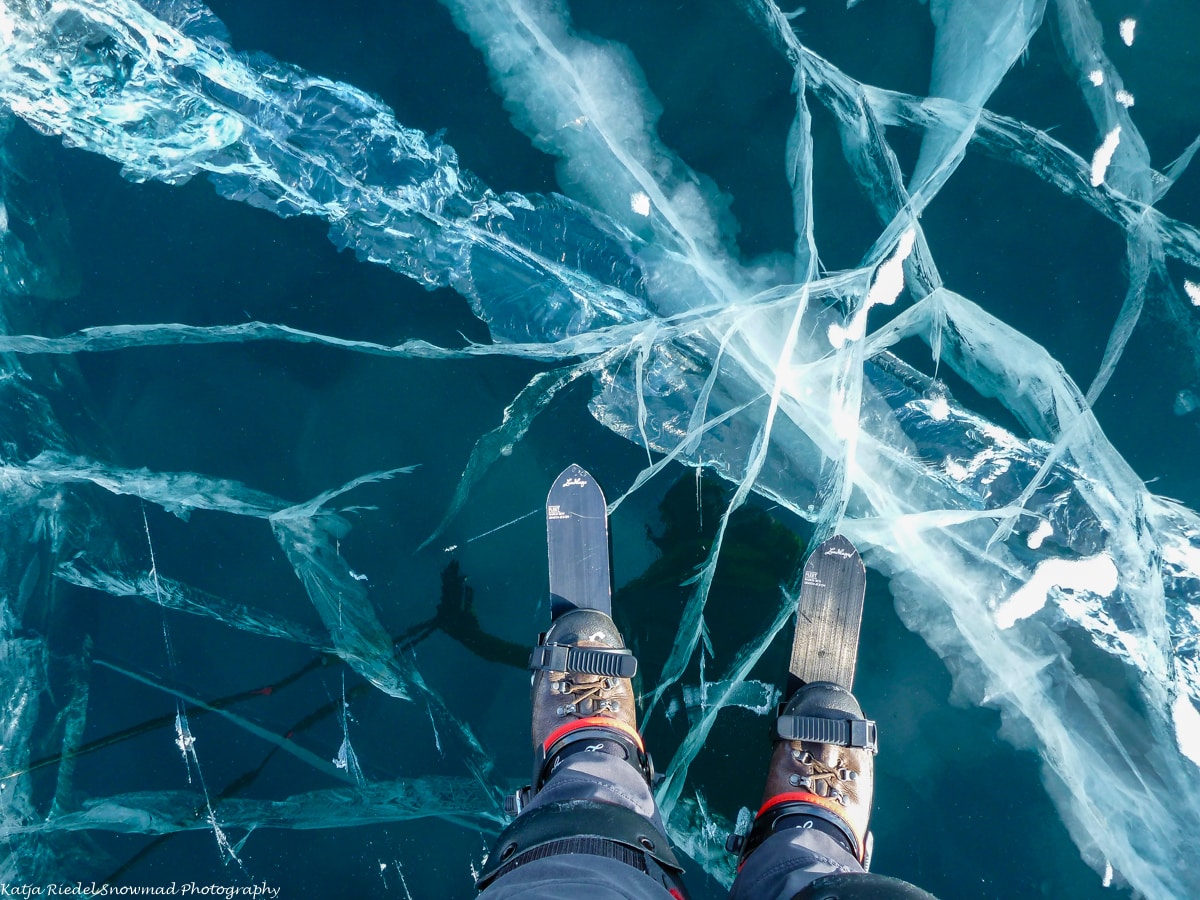In this full-color, outdoor photograph taken during the daytime, a person standing on cracked, reflective ice captures their own image. The photo, square-shaped with no border, reveals a cold, natural setting dominated by blues and whites. The scene is punctuated by the photographer's reflection on the ice, which is riddled with large, intricate cracks. The individual wears brown boots with yellow laces and orange accents, secured into tiny skis that extend just inches beyond their toes. They are also dressed in blue pants and are holding poles, indicating a snowshoeing or ski-touring activity. The detailed textures of the fractured ice emphasize the precarious nature of the surface. The lower left corner of the photo features the text "Katcha Rydell Snomad Photography," underscoring the professional and adventurous spirit of the image.